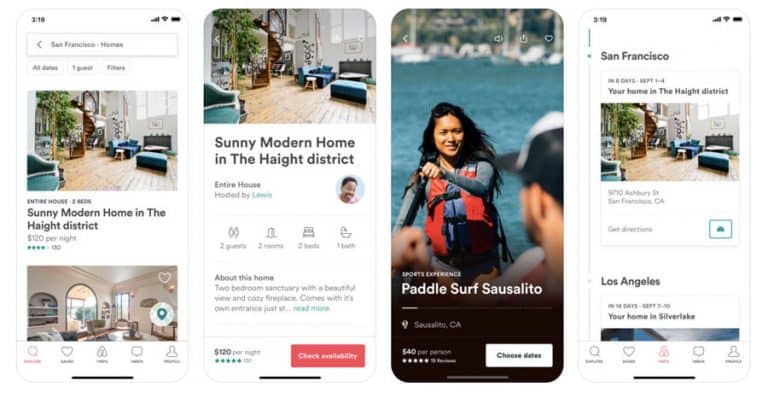This series of four screenshots depicts images displayed on a smartphone screen. Three of the screenshots showcase the same image: a sunny, modern home located in the Heights district, featuring wood floors and minimalist furnishings. The fourth screenshot diverges, showing a picture of a woman in a life vest with the text "Paddle Surf Sausalito," along with an option to select dates. Each screenshot displays the same website at different instances, evidenced by the timestamp of 3:19, as well as visible Wi-Fi and battery icons. The purpose of the varied displays seems to be to compare different aspects of the website's presentation.